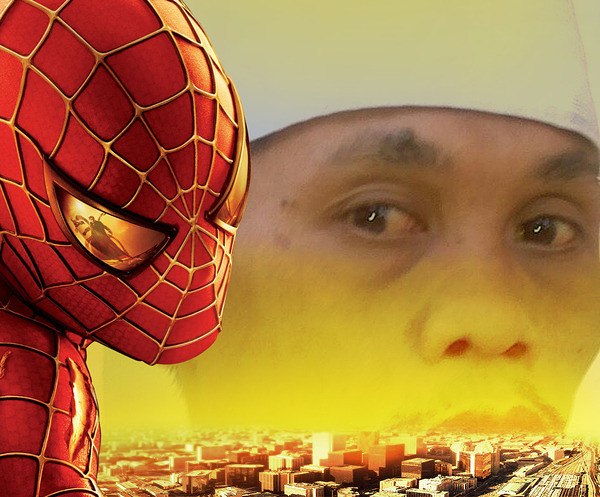The image features a striking foreground of Spider-Man, showcasing only his face and a portion of his shoulder. Spider-Man sports his iconic red suit, adorned with intricate golden webbing. His mask features large eyes edged in black with metallic golden outlines, and in his left eye, there is a reflection of the villain Doc Ock, recognizable by his tentacles. Behind Spider-Man, the background presents a blend of elements: a translucent face of an Asian person wearing a white headgear, which appears to be looking at Spider-Man. Below this face, the background transitions into a golden sky, resembling a sunset, and further down, a detailed cityscape with numerous high-rise buildings and a potential train depot on the right side. The perspective renders Spider-Man as a dominating figure, significantly larger compared to the distant city below, creating a dramatic and heroic visual composition.